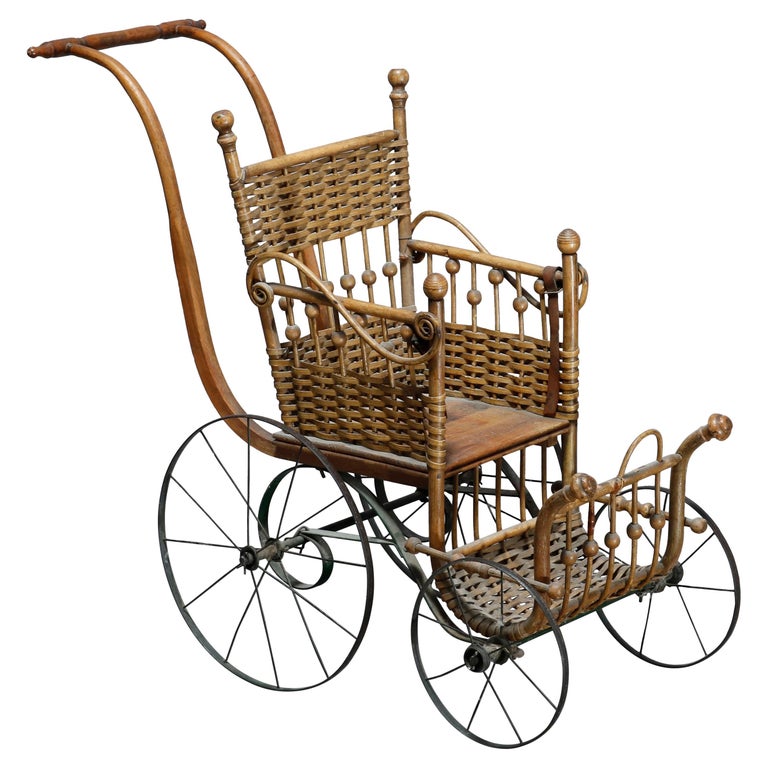This detailed image is a photographic-style depiction of a vintage Victorian wicker wheelchair or baby carriage set against a stark white background, giving it a floating appearance. The carriage features a mix of materials and intricate design elements. The chair showcases a woven wicker backrest, sides, and footrest, suggesting meticulous craftsmanship. Its seat appears relatively large, further suggesting it might function as a wheelchair rather than just a baby carriage.

The design includes four slender metal wheels with iron spokes radiating from central hubs. Interestingly, the front wheels are smaller than the back ones, enhancing its distinctive look. Wooden elements are present in the form of dual curved handles and a middle handle between the wooden bars, which allows for easy maneuvering of the cart. The chair is supported by four posts, each capped with a knob.

There are no texts or inscriptions visible in the image, keeping the focus solely on the detailed and nostalgic design of the vintage carriage.